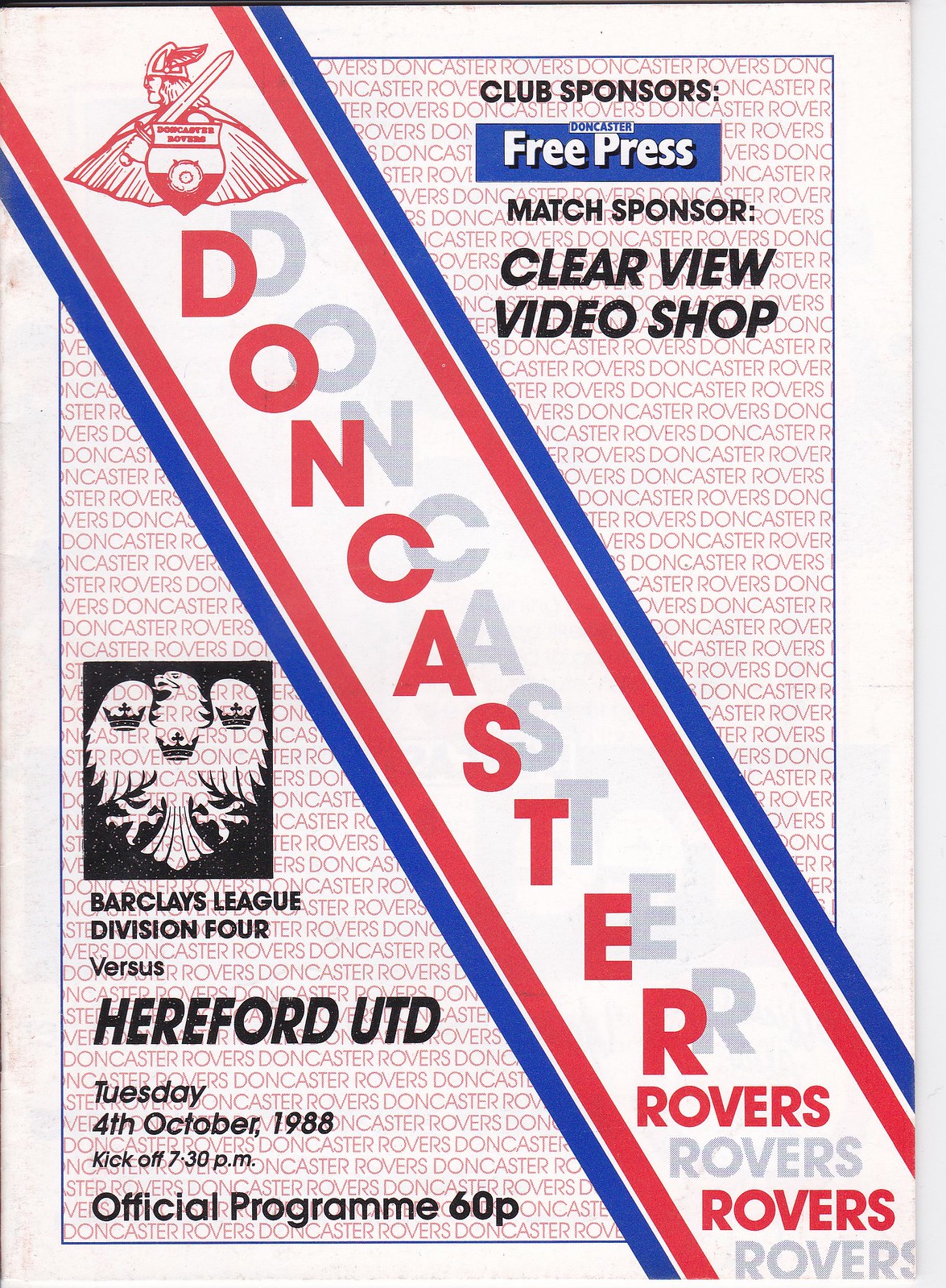This is the 1988 October front cover of an official match program for the Doncaster Rovers, a football club from the Barclays League Division 4. The cover features an intricate and ambitious design on a white background with an additional white border. A significant red and blue bordered diagonal stripe extends from the top left to the bottom right, prominently displaying the club name "Doncaster Rovers" in red. 

Overlaying this pattern in the upper right corner are the club and match sponsors listed in black, blue, and white text, including the Doncaster Free Press and the Clearview Window Shop. A faint and repetitive pattern of "Doncaster Rovers" in small red print further decorates the background within the white border, adding a detailed texture.

On the bottom left sits an image of three birds underlined with the text "Barclay League Division 4" in black, paired with the match information "versus Hereford UTD, Tuesday 4th October 1988, kickoff 7:30 p.m." Also noted is the program's price, "Official Program 60p." The design melds red, blue, and black colors to create a dynamic and historic presentation.